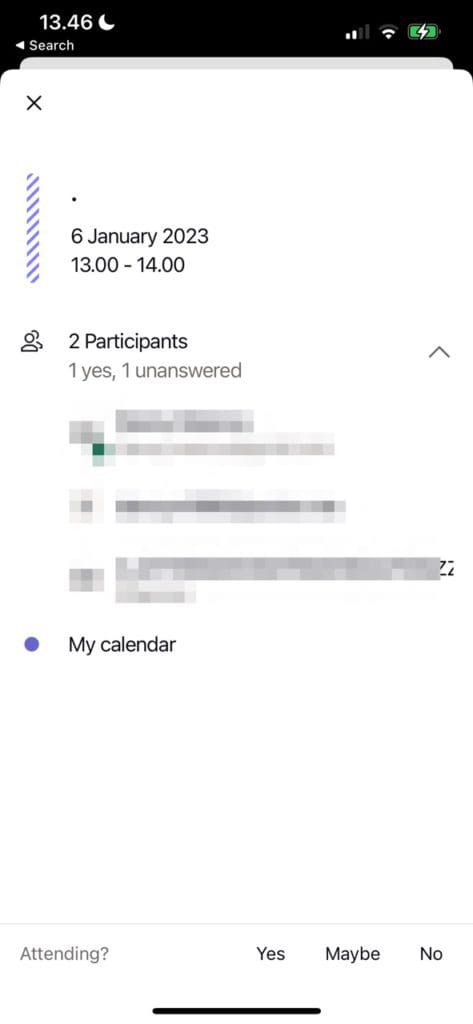The image is a screenshot from a cell phone displaying event details from a calendar app. Against a black toolbar at the top, the time 13:46 and a moon icon indicate it is nighttime. The phone shows two out of four bars of data signal, two out of three bars of Wi-Fi signal, and the battery is fully charged. 

On a white background, the event is scheduled for 6 January 2023 from 13:00 to 14:00. It notes that there are two participants: one has responded 'yes,' while the other has not answered. Three sections of the image are intentionally blurred to protect sensitive information. Below these sections, a blue dot aligns with the text "My Calendar," signifying the calendar source. Further details include an "Attending" section, marked with a question mark, and response options listed as 'Yes,' 'Maybe,' and 'No' in varying text colors.

This screenshot captures the interface of a calendar app, illustrating participant responses and event specifics.